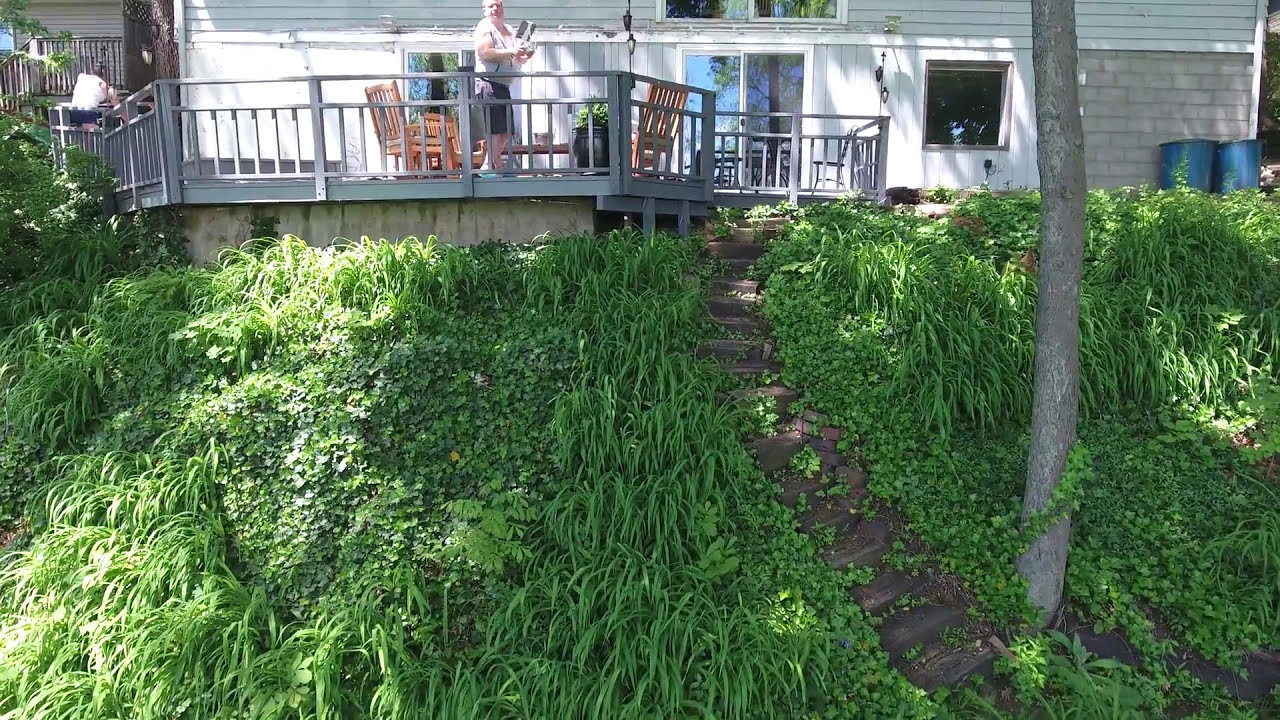The image depicts a white house situated atop a steep, grassy hill abundant with vegetation and weeds. A small, wooden stepped pathway, partially overgrown with grass, leads up the hill to a gray-painted deck on the backside of the house. The deck, bathed in bright sunlight, reveals a man standing near the center, straightening up from a patio chair and clutching a couple of books or a laptop to his chest. There is a closed sliding patio door, flanked by two square windows, that opens onto the deck from the house. On the far left side of the deck, another man is perched on the railing. The deck is adorned with several chairs and a table, and there are two garbage cans positioned against the rear wall of the house. A skinny gray tree stands in front, with its shadows cast prominently in the sunlight.